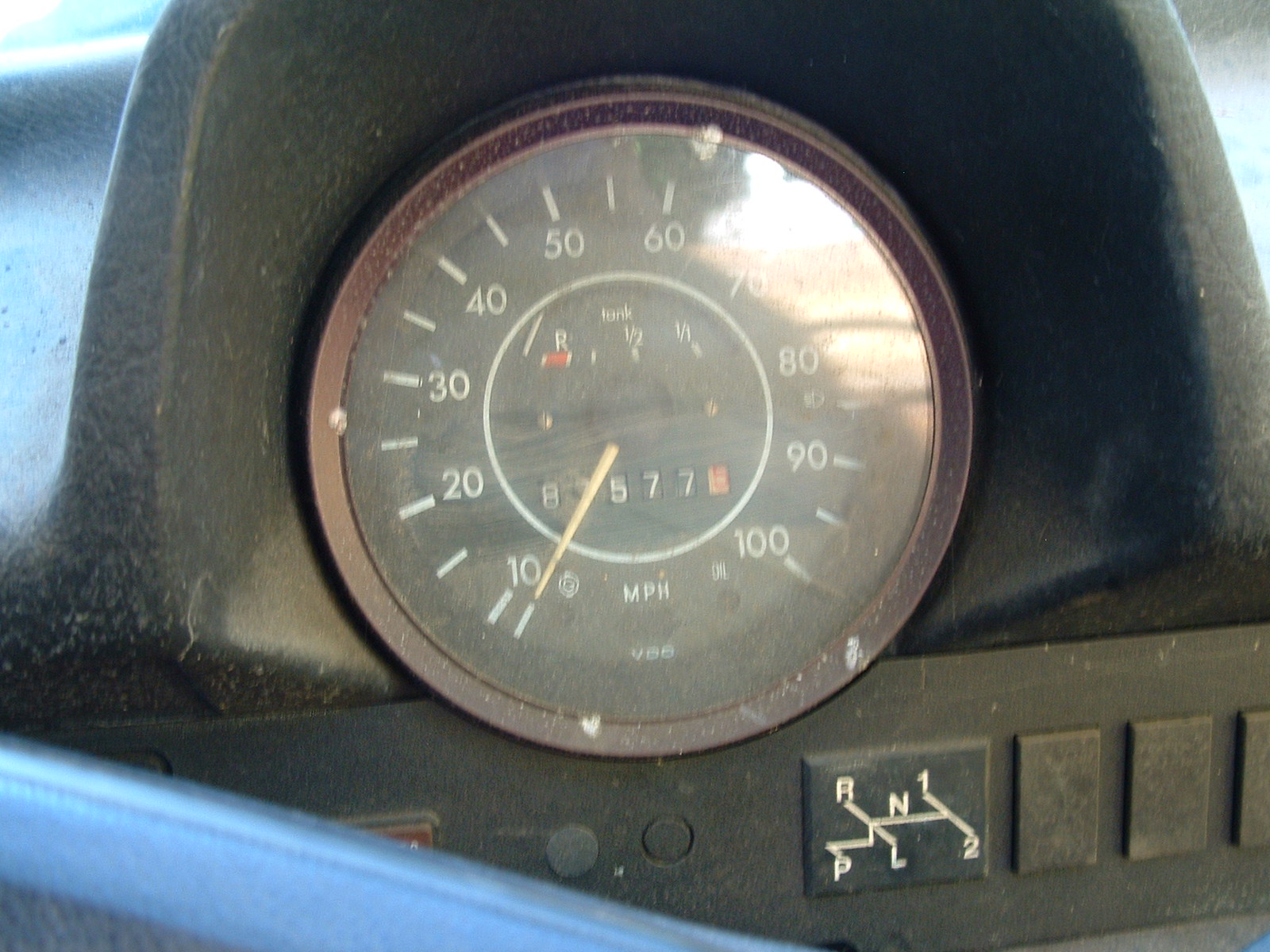A detailed close-up photo captures a vintage speedometer encased in a round frame with a brownish outer ring. The speedometer has a clear lens on top and features white dashes circling its face. Every other dash is marked with a number in increments of 10, starting from 10 and continuing up to 100. Below the numbers, two small black nubs protrude from the plastic casing.

To the right side of the speedometer, there is a black square display showing gear indicators labeled with "R, P, L, N, 1, 2," connected by a series of lines demonstrating the gear transition paths: a line between 1 and 2, another connecting L and R, one line linking N above, and a final line connecting P below. These gear positions likely stand for Park, Reverse, Neutral, Low, and forward gears 1 and 2.

The entire speedometer is set within a black recessed area adding depth to its placement. The dial contains several inscriptions: "8, 5, 7, 7, tank, R," with the letter 'R' highlighted in red. Additional markings showing "dash mark, 1, 1" appear on one half of the dial, and at the bottom, the speedometer is labeled "MPH V88."